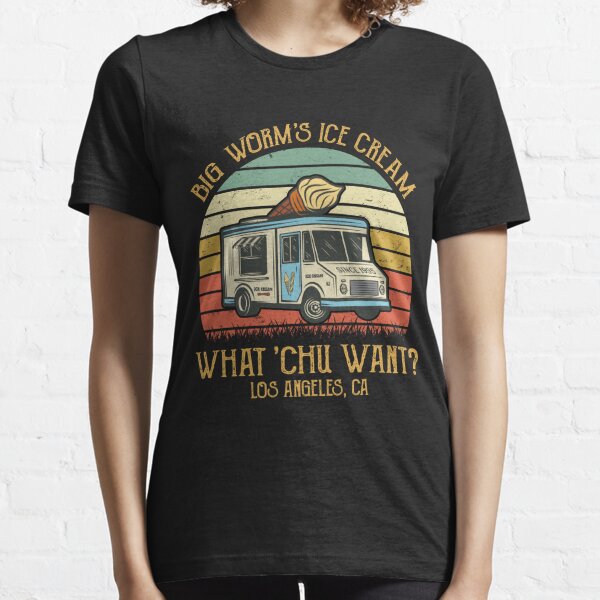The image features a person standing against a white wall with a brick pattern, dressed in a black t-shirt and black pants. The photo is cut off just above the person's neck, and also cut off below the waist, rendering the person's hands invisible at their sides. The person has fair skin and shoulder-length curly red hair, although their face is not shown.

The black crew neck t-shirt prominently displays a vibrant design in the center, depicting an ice cream truck with a giant ice cream cone on top. The truck is adorned with colorful livery: white and blue with a red bottom, yellow middle, and white top, blending into a blue sky. The scene behind the truck shows abstract patterns in blue, white, yellow, and red, along with a strip of black resembling grass at the base.

Across the top of the design, in yellow text, are the words "Big Worms Ice Cream." Below the illustration, framed by the colors, the text reads "What Chew Want" in a playful, stylized manner, followed by "Los Angeles, CA" below it in smaller text. This detailed and eye-catching t-shirt effectively captures the whimsical spirit of the Big Worms Ice Cream brand.